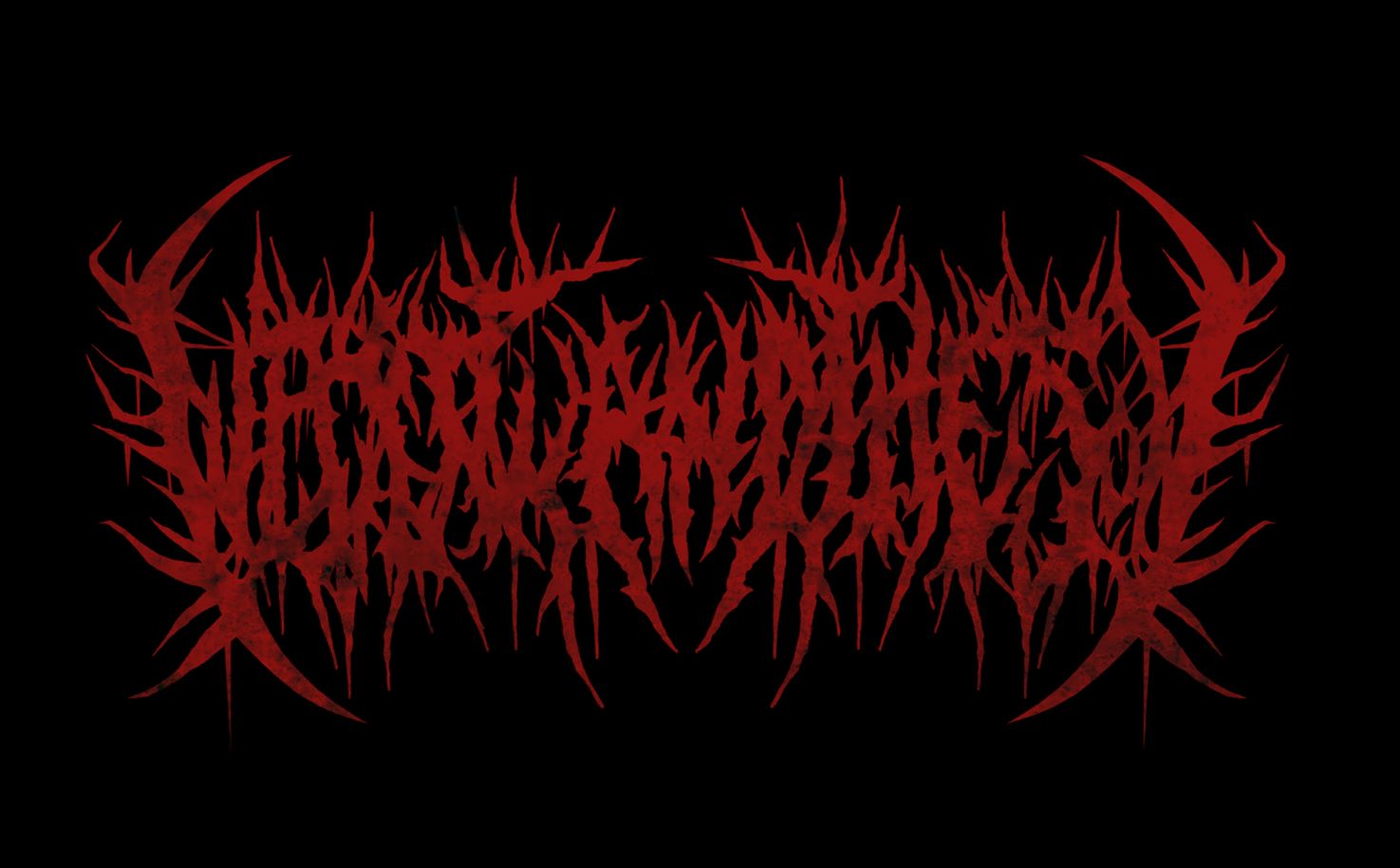The image features a striking, abstract graphic set within a horizontal rectangular frame, twice as wide as it is tall. The background is a solid black, providing a stark contrast to the crimson elements in the center. Dominating the middle of the image is an intricate, dense formation of jagged, thorn-like shapes that resemble a tangle of brambles or jagged sticks. These sharp, blade-like red forms are splotchy and give the impression of dripping red paint, heightening their vivid, almost menacing appearance. The overall effect is a vivid red mass of thorns with longer spikes on the left and right edges, and shorter, equally pointed thorns in the center. The graphic has a chaotic, almost visceral quality, as if capturing the essence of sharpness and danger amidst a stark, dark void.